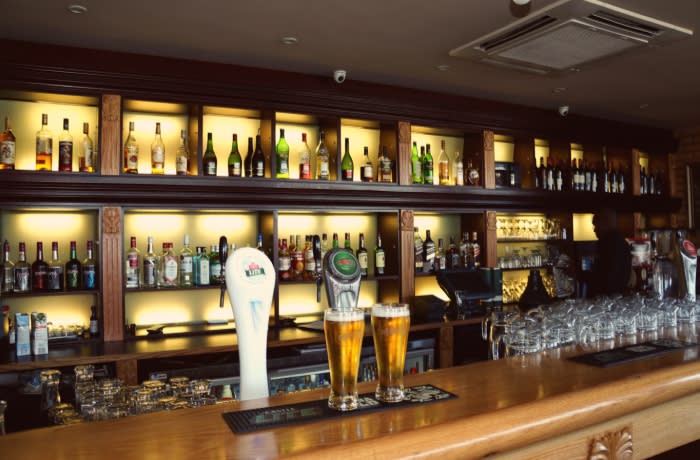This photograph captures an empty bar from the customer's perspective, showcasing a light honeywood bar top with two full pint glasses of beer prominently placed on it. Behind the bar, a dark brown wooden back display stretches the entire width of the image. This display features rows of illuminated shelves, each housing neatly arranged bottles of alcohol. The top row consists of smaller square compartments, each holding three to four bottles, while the larger rectangular compartments below them have horizontal shelves lined with long rows of bottles, all accentuated by warm yellow lighting. To the right behind the bar, there are rows of beer mugs or drink mugs, and to the left, inverted clear pint glasses are visible. The scene is dimly lit, though the illuminated compartments behind the bar cast a gentle glow on the array of bottles. Above, a light gray ceiling features a large rectangular light on the right side and several white security cameras positioned along the back.